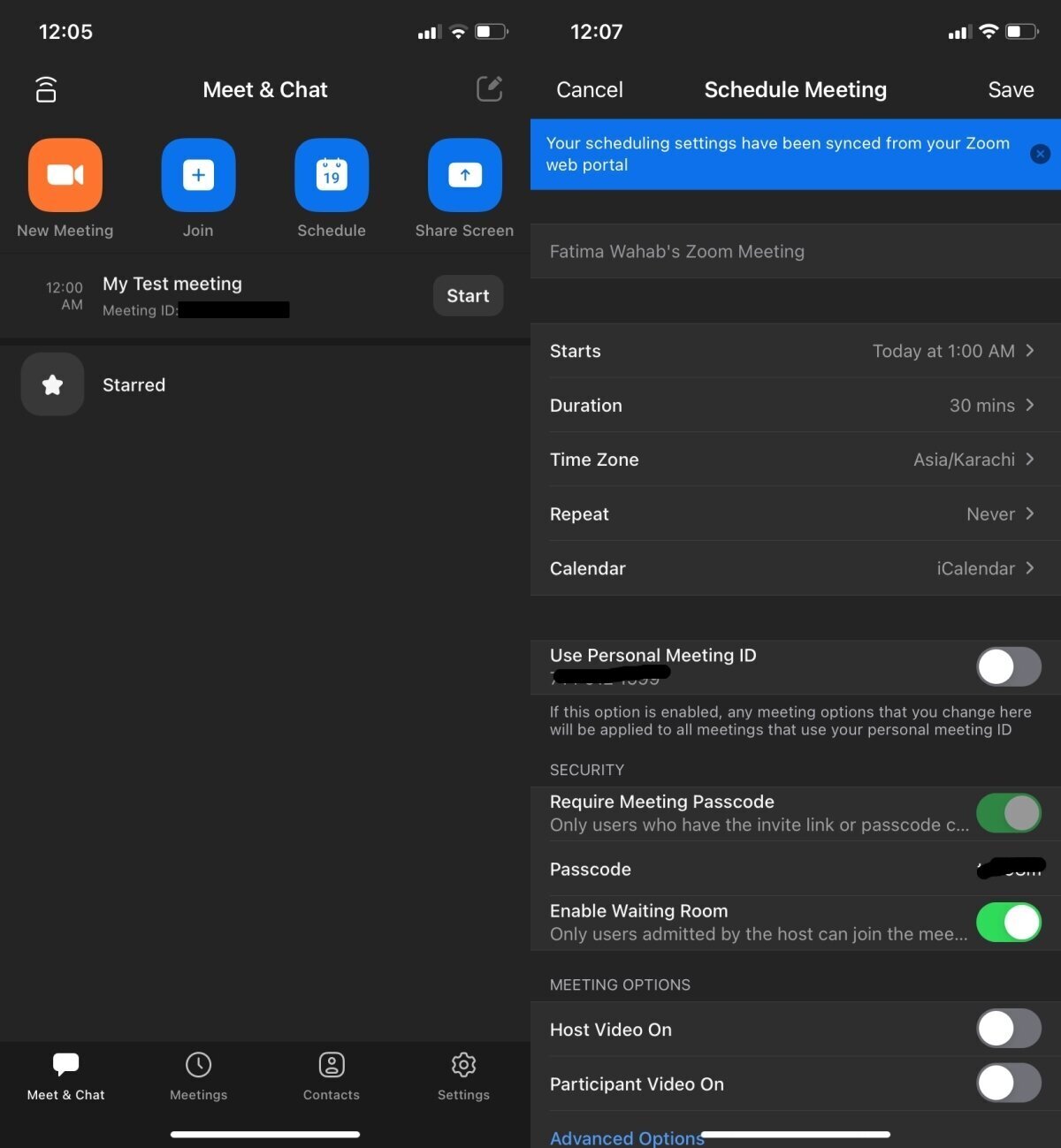The image displays two screenshots side by side, captured from a cell phone, as evidenced by the visible status bar at the top, complete with the clock, signal strength, and battery meter. 

The left screenshot features a "Meet & Chat" interface. Prominently at the top are clickable buttons or icons for "New Meeting," "Join," "Schedule," "Share," and "Share Screen." Below these options is a section labeled "My Test Meeting," accompanied by a "Start" button, indicating an ongoing or scheduled meeting.

The screenshot on the right showcases the synchronization of scheduling settings from the Zoom web portal. It highlights a meeting organized by Fatima Wahab. Details include:
- "Starts: Today at 1 AM"
- "Duration: 30 minutes"
- "Time Zone: Asia/Karachi"
- "Repeat: Never"
- "Calendar: iCalendar"

Additionally, the settings display toggles for various preferences, such as:
- "Use Personal Meeting ID" (turned off)
- "Require Meeting Passcode" (turned on)
- "Enable Waiting Room" (turned on)

Lastly, there are options regarding video settings, with "Host Video On" and "Participant Video On," both set to off.